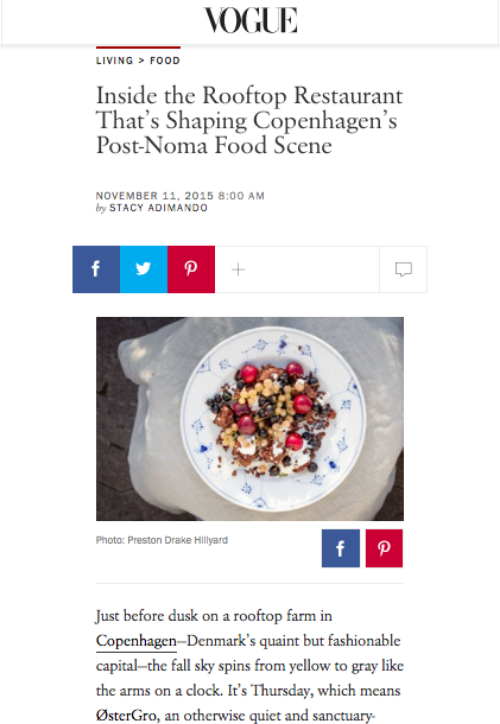From the Vogue online magazine's "Living" section, specifically under "Food," a captivating article titled "Inside the Rooftop Restaurant That’s Shaping Copenhagen’s Post-Noma Food Scene" was published on November 11, 2015, at 8 a.m. by Stacey Adamondo. This piece, available for sharing on Facebook, Twitter, and Pinterest, and open for comments, features a visually intriguing dish. The image shows a beautifully presented meal in a pristine white porcelain bowl nested inside a larger, irregularly-shaped glass dish, reminiscent of jelly. The dish includes a medley of beans, a dollop of sour cream or a similar creamy element, corn, and tomatoes, among other fresh ingredients. The caption beside the dish reads: "Just before dusk on a rooftop farm in Copenhagen, Denmark's quaint but fashionable capital, the fall sky spins from yellow to gray like the arms on a clock. It’s Thursday, which means Ostergrove, an otherwise quiet sanctuary, becomes a hive of activity centered around locally-grown produce. The meal looks healthful, though one might find themselves wanting more."